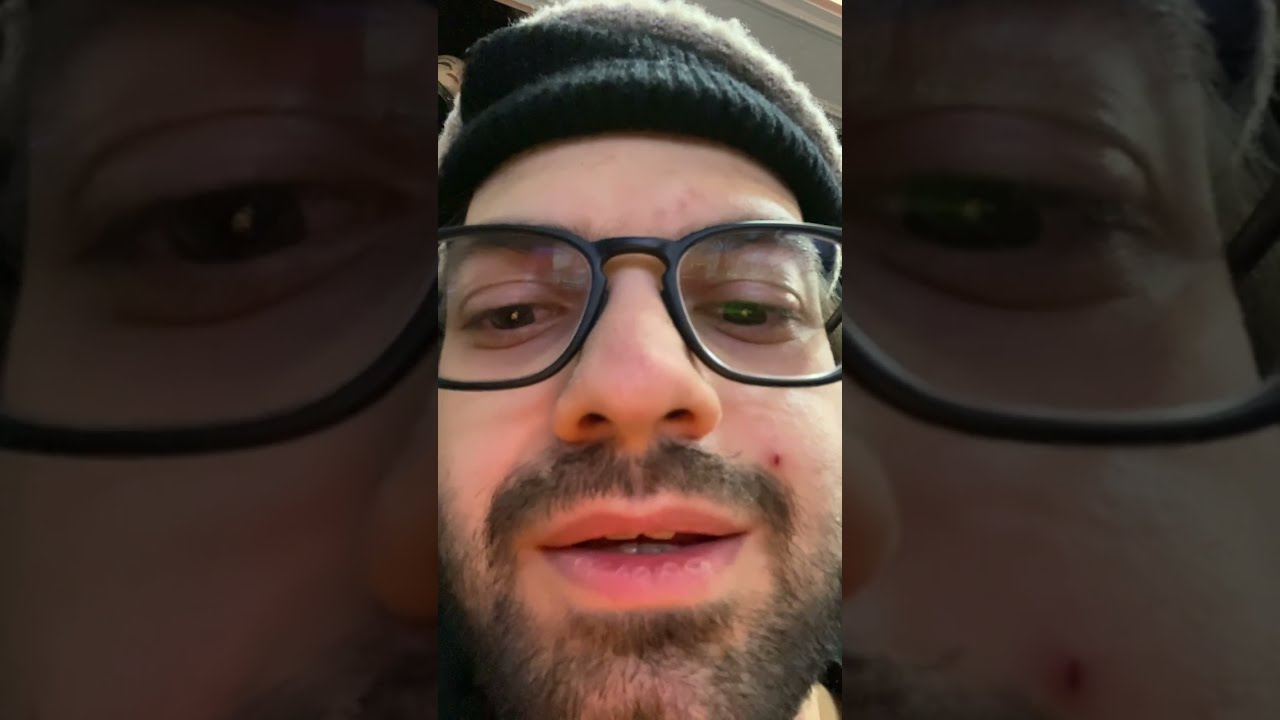The image is a composite image split into three sections. The central section is an up-close selfie of a white man wearing a black beanie, black round glasses, and a thin black goatee. He has a slightly brownish-black beard and mustache. He appears to be smiling and looking down, with a small zit visible on his left cheek. The background is a gray-toned storefront with light gray molding, suggesting the photo was taken outside. The left and right sections are zoomed-in, darkened excerpts of the same image, focusing respectively on the left and right sides of the man’s face. The left section shows his left eye, partial mustache, and the bottom rim of his glasses, while the right section mirrors this with his right eye and similar facial features. The sunlight reflects off his glasses, and the entire composition hints at a cold day, possibly due to the beanie he is wearing.